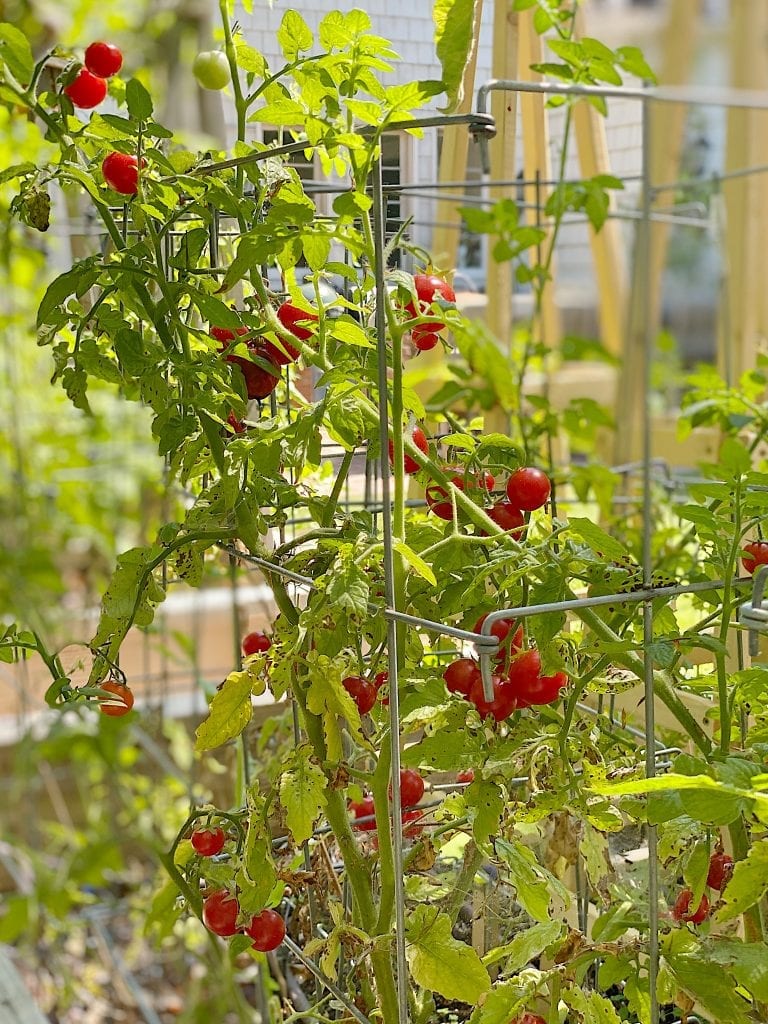This photograph captures a vibrant garden scene on a bright, sunny day, with the focal point being multiple cherry tomato plants. The tomato plants are supported by a metal wire structure to keep them upright. These plants are laden with numerous small, round tomatoes, predominantly ripe and deep red, though some are still a light green and yet to ripen. Despite their bounty, the plants exhibit considerable leaf damage, with noticeable browning among the bright green foliage. In the blurred background, other garden plants and a white house with visible windows add depth to the scene. The intricate details of the garden, combined with the lush, sunlit surroundings, suggest a well-tended, albeit slightly struggling, tomato patch in a residential setting.